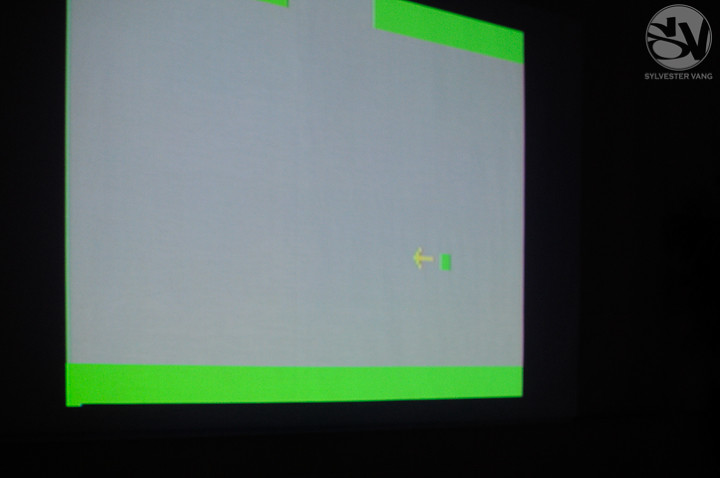A meticulously designed graphic image, potentially created for a corporate project or a computer game, prominently features the name "Sylvester Vang" aligned to the right. The central square hosts a fluorescent green line traversing a portion of its top edge. A distinct lime green arrow points towards a small lime green square or rectangle, adding dynamic visual interest to the layout. At the bottom, a lime green horizontal line stretches from side to side, complementing the color scheme dominated by gray and lime green elements against a stark black background. The structured elements and vibrant colors suggest that this image is a part of a professional project or a creative endeavor in progress.